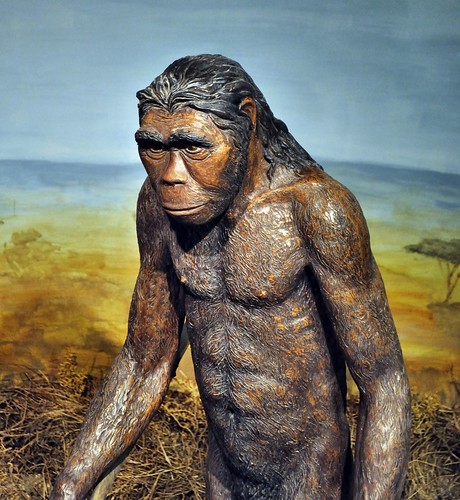The photograph captures a detailed statue of a prehistoric humanoid, presumably displayed in a museum of science and history. This statue depicts a stereotypical heavy-browed male with a broad nose and forehead, a characteristic thin chest, and long, dark hair. The figure is covered in a light coat of fur and features thick eyebrows, a prominent beard, and discernibly hairy arms and chest. The humanoid's skin tone is a medium brown, and the stance suggests he's mid-step, adding a dynamic element to the sculpture.

In the background, a painted backdrop showcases an African savannah under a clear blue sky. The watercolor-style painting includes details such as a prominent baobab tree on the right-hand side and an array of dried grasses and straws, enhancing the prehistoric theme of the display. The overall setting resembles a scene from the African plains, providing a contextual and immersive environment for the statue.